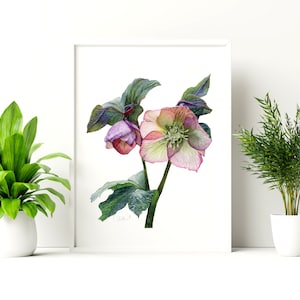In this photograph, the central focus is a framed watercolor painting of a flower, predominantly featuring dark green leaves with petals in various shades of pink and light lavender, and a green center. The painting is set against a clean, white background and shadowed subtly behind the frame, which also contrasts against the white wall. Flanking the painting, there are two small potted plants in white ceramic pots. The plant on the left has larger, brighter leaves that resemble those of an aloe, while the plant on the right has smaller, darker branches with bushier, spikier leaves. The entire scene is set against a pristine white surface that forms the floor of the image.